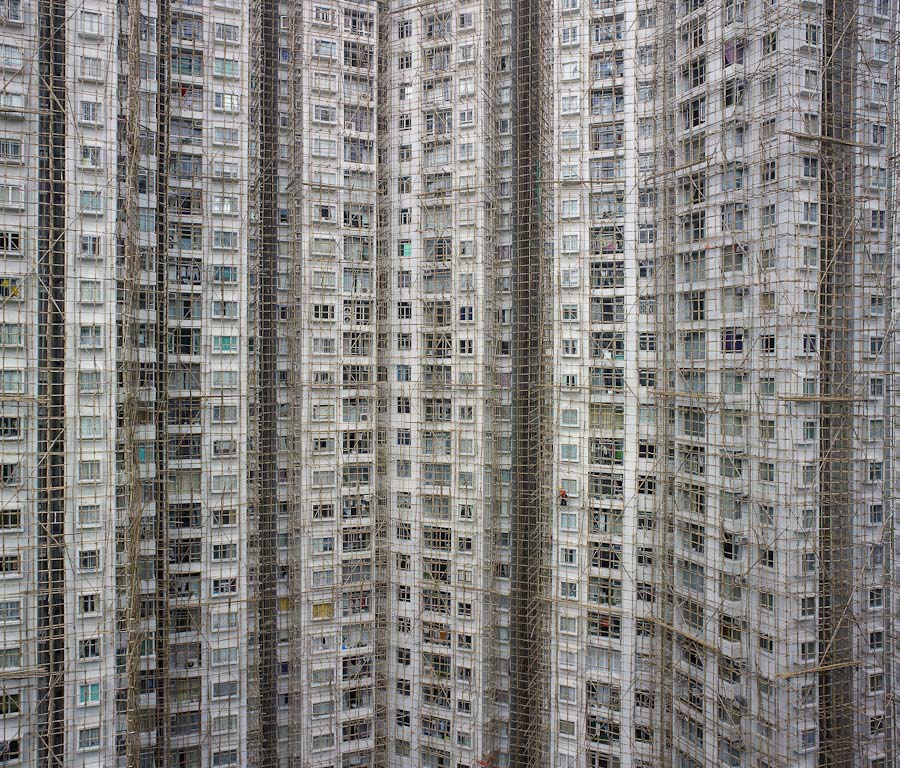This photograph captures a massive high-rise complex, possibly an apartment building in a developing country. The image is focused on approximately 17 to 18 floors, with numerous windows and balconies visible. The structures are predominantly white in color. Surrounding the entire exterior of the building is extensive metal scaffolding, indicating ongoing construction. Wooden planks and a wooden gate-like structure are also seen encasing the building, restricting the view and access from the windows. The photograph seems to have been taken from a considerable distance, revealing a man standing on the scaffolding, adding to the sense of scale and the ongoing nature of the construction work.